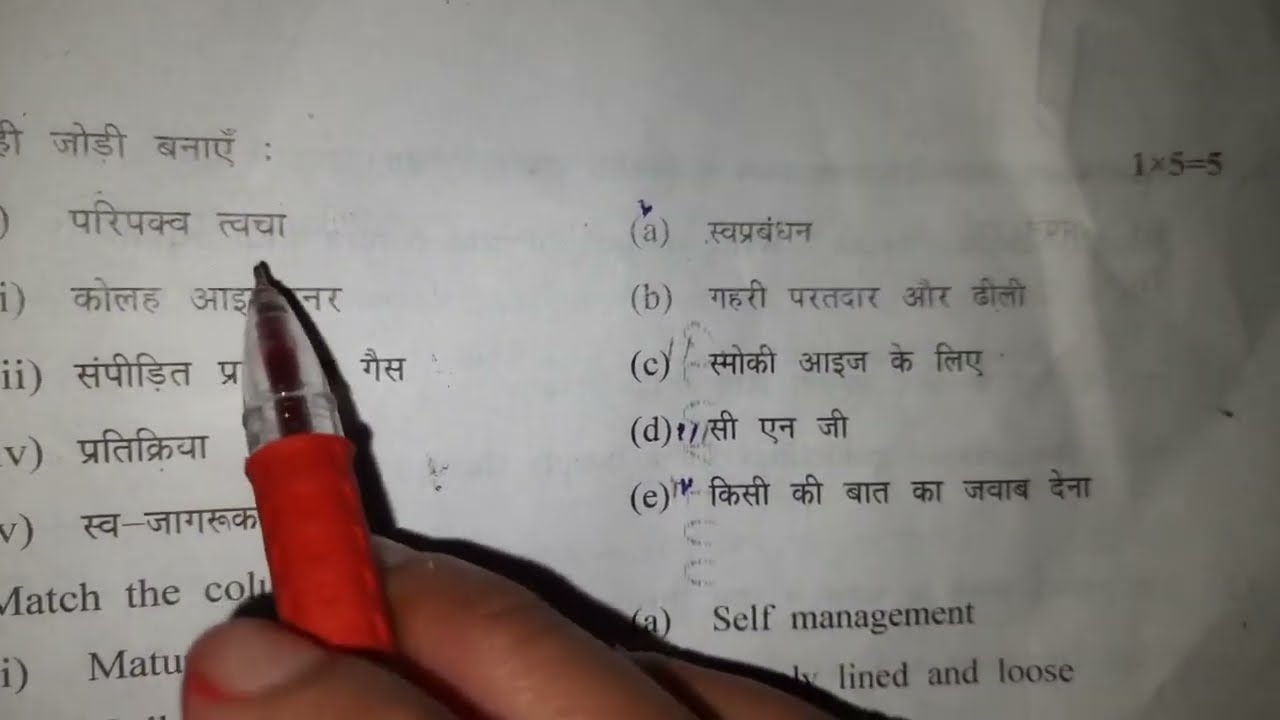The image captures a detailed, close-up photograph of a hand poised above a white sheet of paper covered in text. The paper features two distinct columns: on the left, partially cut-off Roman numerals run vertically alongside eight lines of text, while the right column lists letters A, B, C, and D followed by lines of text in what appears to be an Asian language. A visible math equation, "1 x 5 = 5," and the phrase "self-management lined loose" stand out on the right side of the paper. In the top-left corner, the phrase "match the" is partially visible. A lighter-skinned hand holding an orange-gripped, silver-tipped pen is positioned at the bottom, with three fingers seen at the edge of the image. The pen is angled toward the second line from the top in the left column, suggesting the individual is about to write or point out something specific.